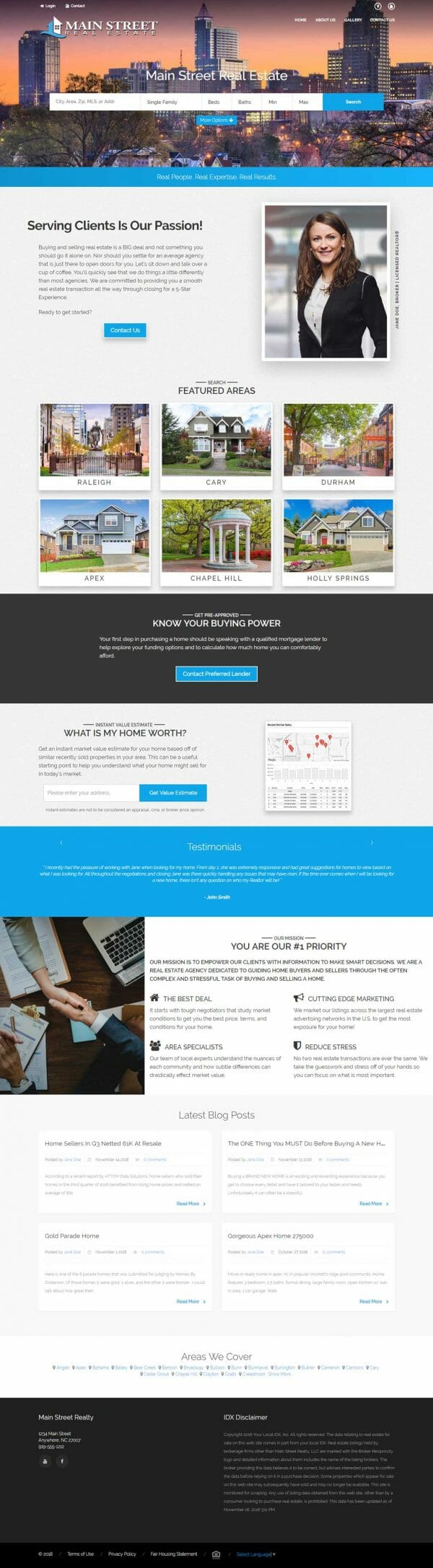In this screenshot captured from a mobile phone display, a user is browsing the Main Street Real Estate website. The header image prominently features a panoramic view of a city, bathed in the warm, gradient hues of a sunset or sunrise, casting the sky in shades of reddish, orangish, and pinkish colors. Below this picturesque vista, blue buttons and links are scattered across the page, emblazoned with a tagline that reads, "Real People, Real Expertise, Real Results."

Centralized on the webpage is a “Contact Us” button, accompanied by a paragraph headed with, "Serving Clients is Our Passion." Continuing to scroll down reveals an image of a professional real estate agent, characterized by her brown hair, black suit jacket, and button-down blouse.

The site also highlights featured areas in and around Raleigh, Cary, Durham, Apex, Chapel Hill, and Holy Springs. There is ample text and navigation options further down, including a section devoted to determining "What Is My Home Worth?" and another emphasizing, "You Are Our Number One Priority."

Towards the middle of the page, the “Latest Blog Post” section showcases four clickable rectangles, and the bottom of the page is filled with small print.